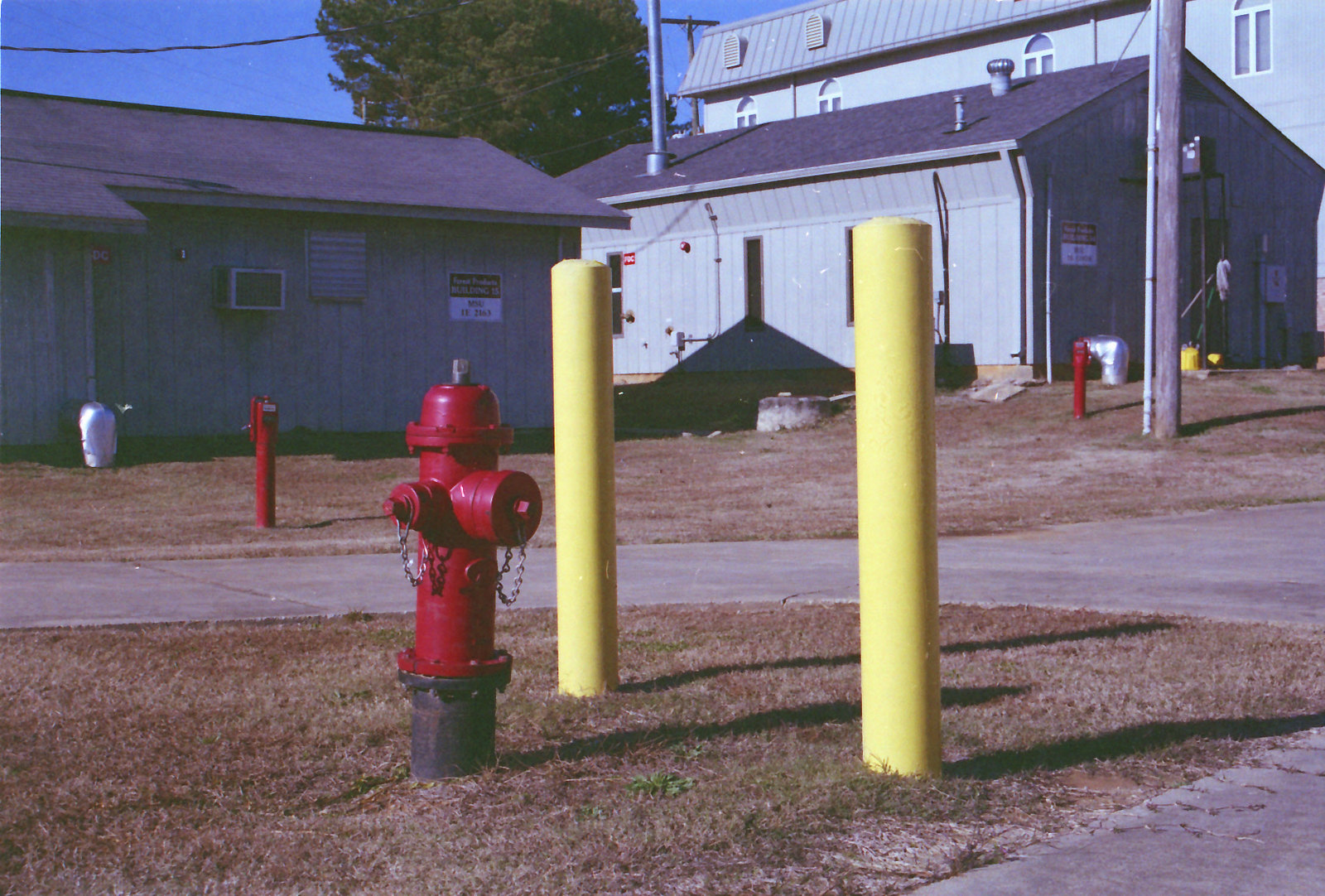In this low-quality outdoor photograph, likely taken with an old Polaroid camera, the scene features three buildings of varying sizes arranged from left to right. The leftmost building sports a red-topped sign with white sections and red lettering, although the specific text is unreadable. Adjacent to it, there's a white trash can. The middle building is slightly wider and has similar signage, with a red sign at the top and a white sign at the bottom, both showcasing unreadable red and white lettering.

The tallest building, situated on the far right, features four windows and roof shutters. A utility pole and power line are visible nearby, along with a large tree that appears subdued due to the setting sun. The foreground includes a red fire hydrant, flanked by two yellow protective poles, casting long shadows onto the ground. The grass around these structures is predominantly brown, indicating it's mostly dead, with just scattered hints of green. Pavement is also visible in the scene, alongside additional red poles and various pieces of safety equipment scattered around the brown grassy area. The buildings in the background, presumably gray manufacturing structures, add to the industrial ambiance of the photograph.